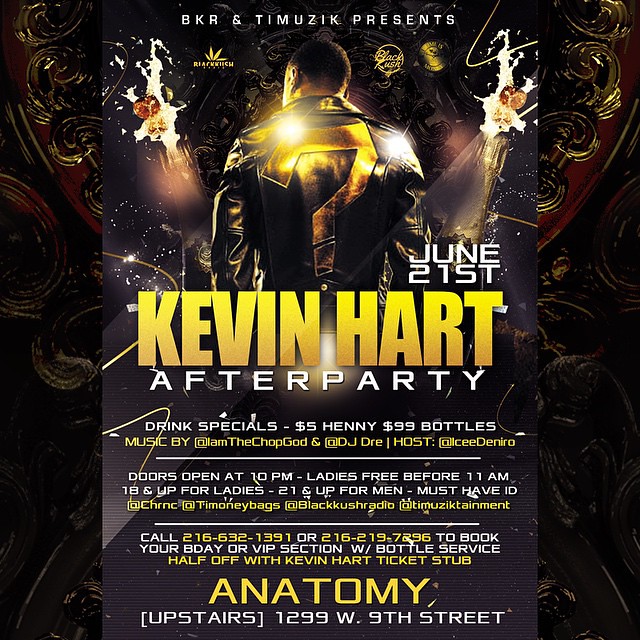This promotional poster for the Kevin Hart After Party, hosted by BKR and Timusic, is a visually striking and detailed design. Set against an ornate black background with glittering energy flares and lens flares, the large yellow-gold text prominently features "Kevin Hart" in the center. Above this, "BKR and Timusic Presents" is written in white, with the event date, June 21st, just below. The central image showcases Kevin Hart from behind, clad in a black leather jacket adorned with a large gold question mark.

The flyer lists drink specials including $5 Henny and $99 bottles, with doors opening at 10 PM. Ladies can enter for free before 11 AM. The event is 18+ for ladies and 21+ for men, with a valid ID required for entry. Contact numbers for booking a birthday or VIP section are provided: 216-632-1391 and 216-219-27296. Special promotions include half-off with a Kevin Hart ticket stub. The venue is the Anatomy Club, specifically the upstairs area, located at 1299 West 9th Street.

Logos and icons such as a weed plant, a gold circled logo, and champagne bottles popping on either side of Kevin Hart add to the poster's opulent feel. The names of the involved personnel and contributors, such as Music by EM The Chop God, DJ Dre, and Host Icy Gennaro, are also featured in various text colors, enhancing the dynamic and festive vibe of the flyer.